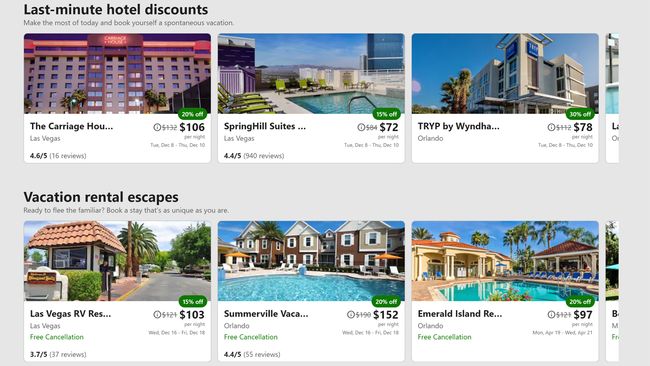This horizontal rectangular image has a light gray background with two rows of smaller horizontal rectangular images. At the top of the light gray area, black text reads, "Last-Minute Hotel Discounts." Below this, smaller black text states, "Make the most of today and book yourself a spontaneous vacation."

### Top Row:
1. **First Image:**
   - **Visual:** A hotel
   - **Label:** "The Carriage HOU"
   - **Price:** $106
   - **Discount:** A green oval with "20% off" in lighter font
   - **Rating:** 4.6/5 (16 reviews)

2. **Second Image:**
   - **Visual:** A swimming pool
   - **Label:** "Spring Hill Suites"
   - **Location:** Las Vegas
   - **Rating:** 4.4/5 (specific number of reviews unreadable)
   - **Price:** $72
   - **Discount:** A green oval with "15% off" in lighter font

3. **Third Image:**
   - **Visual:** The exterior of a hotel
   - **Label:** "TRYP by Wyndham"
   - **Location:** Orlando
   - **Price:** $78
   - **Discount:** A green oval with "30% off"

4. **Fourth Image:**
   - **Visual:** Partially visible, a cut-off image.

### Bottom Row:
- The heading reads "Vacation Rental Escapes"
- Below it, small text states, "Ready to flee the familiar? Book a stay that's as unique as you are."

1. **First Image:**
   - **Visual:** A tropical area with palm trees
   - **Label:** "Las Vegas RV" (cut off)
   - **Location:** Las Vegas
   - **Cancellation Policy:** Green text, "Free cancellation"
   - **Rating:** 3.7/5 (37 reviews)
   - **Price:** $103
   - **Discount:** A green oval with "15% off"

2. **Second Image:**
   - **Visual:** What looks like three townhouses with a beautiful pool in front
   - **Label:** "Somerville Vacay"
   - **Location:** Orlando
   - **Cancellation Policy:** Green text, "Free cancellation"
   - **Rating:** 4.4/5 (55 reviews)
   - **Price:** $152
   - **Discount:** A green oval with "20% off"

3. **Third Image:**
   - **Visual:** A pool area with blue chairs around the pool and open-air buildings
   - **Label:** "Emerald Island"
   - **Location:** Orlando
   - **Cancellation Policy:** Green text, "Free cancellation"
   - **Price:** $97
   - **Discount:** A green oval with "20% off"

4. **Fourth Image:**
   - **Visual:** Partially visible, a cut-off image.